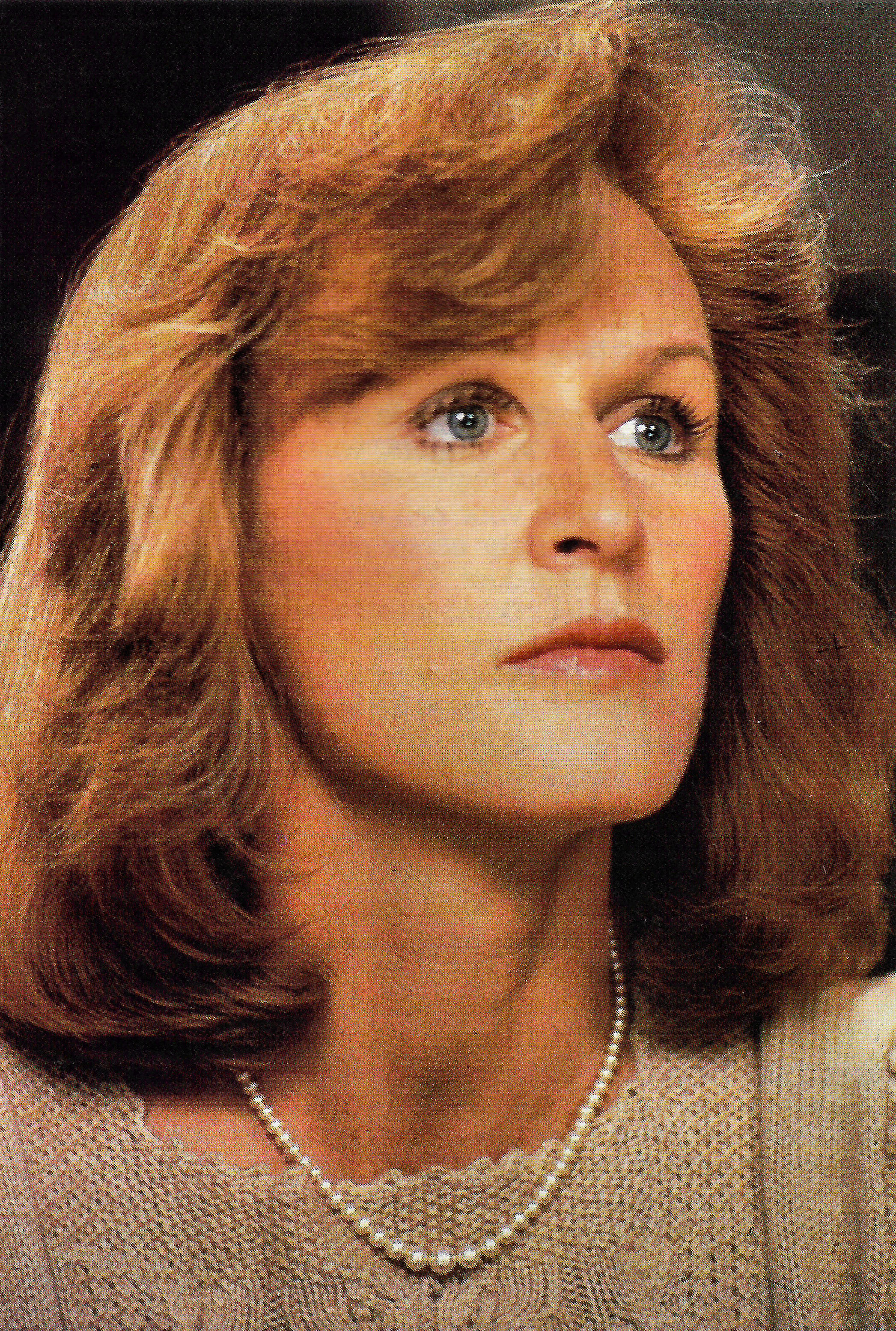The image depicts a middle-aged woman viewed from the shoulders up, with a hairstyle characteristic of the 70s or 80s. She has a feathered, slightly wavy dirty blonde hair that falls to her shoulders, and she sports bangs that partially cover her high forehead. Her hair catches some highlights from the lighting, giving it a nuanced tone between light brown and auburn. She wears a cream-colored knit sweater adorned with different cable and stitch patterns, complemented by a string of pearls that rests just above the sweater's neckline. Her makeup is subtle, featuring black mascara, eyeliner, blush, and a pinkish-red lip color. She has bluish-green eyes and dark eyebrows. Captured with an inquisitive or intense expression, she looks slightly up and to the left, her small nose and the lighting emphasizing her intrigued demeanor.